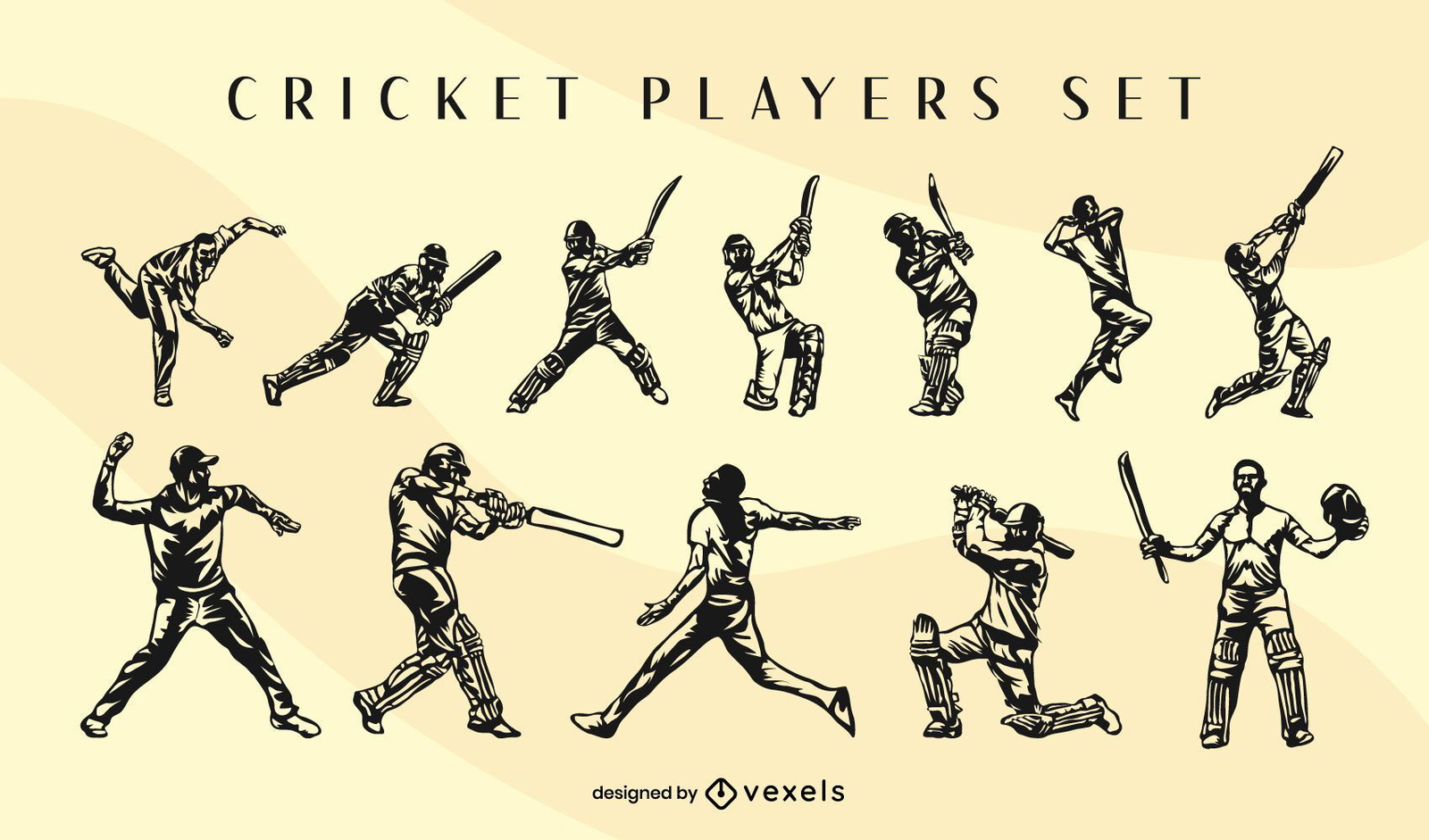The image is a detailed poster titled "Cricket Player Set" in black, uppercase font centered at the top. The background is a pale yellow with a subtle, swirly pattern. The drawing features 14 cricket players depicted in black ink, arranged in two rows. The top row consists of seven action figures, showing different stages of gameplay, such as pitching, swinging a bat, and preparing to bat. Notably, the first player appears to be leaning forward in a pitching stance, while the last player holds the bat upright. The second row, featuring slightly taller figures, displays five players in various actions, including pitching, batting with protective gear like helmets and shin guards, running, and kneeling with a bat. At the bottom center, the text "Designed By Vexels" is written in smaller black font, separated by a diamond-shaped icon.